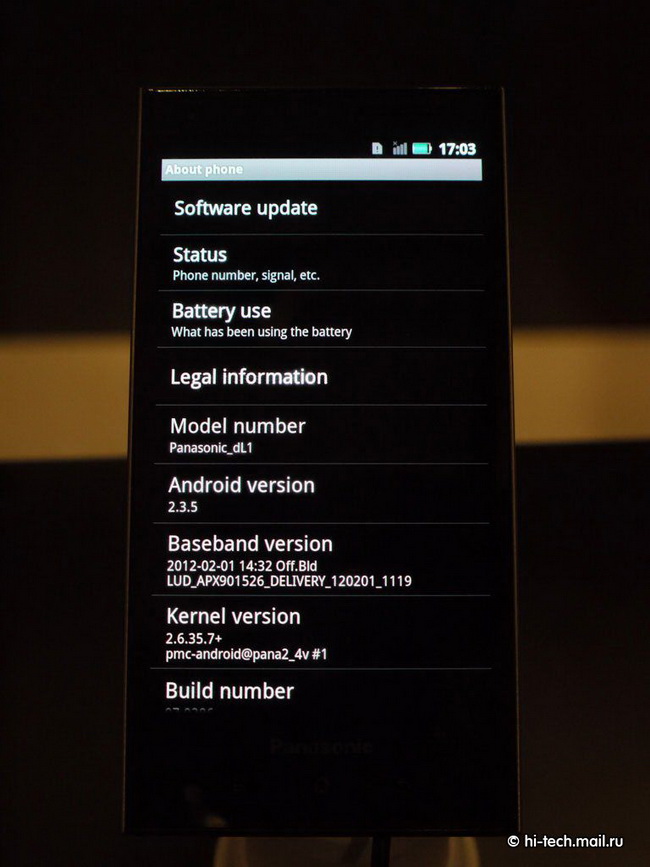The image displays a smartphone showcased on a stand with a dark background and a stripe of blurry gold or yellow behind it. The phone screen shows the "About Phone" menu of an Android device, displaying details in white text against a black background. The status bar at the top reveals the time as 17:03, a nearly full green battery icon, and symbols denoting internet connection and signal strength. The "About Phone" menu includes several items: 

1. **Software Update**
2. **Status**
3. **Phone Number**
4. **Signal, etc.**
5. **Battery Use** - detailing what has been using the battery.
6. **Legal Information**
7. **Model Number**: Panasonic_DL1
8. **Android Version**: 2.3.5 
9. **Baseband Version**: 2012.02.01.14.32 off BLD
10. **Kernel Version**: 2.6.35.7+ PMC-Android@Pana2_4V#1

Though the build number is also mentioned on the screen, it's not visible due to the need for scrolling. In the bottom right corner, the copyright notice "hightech.mail.ru" is displayed.